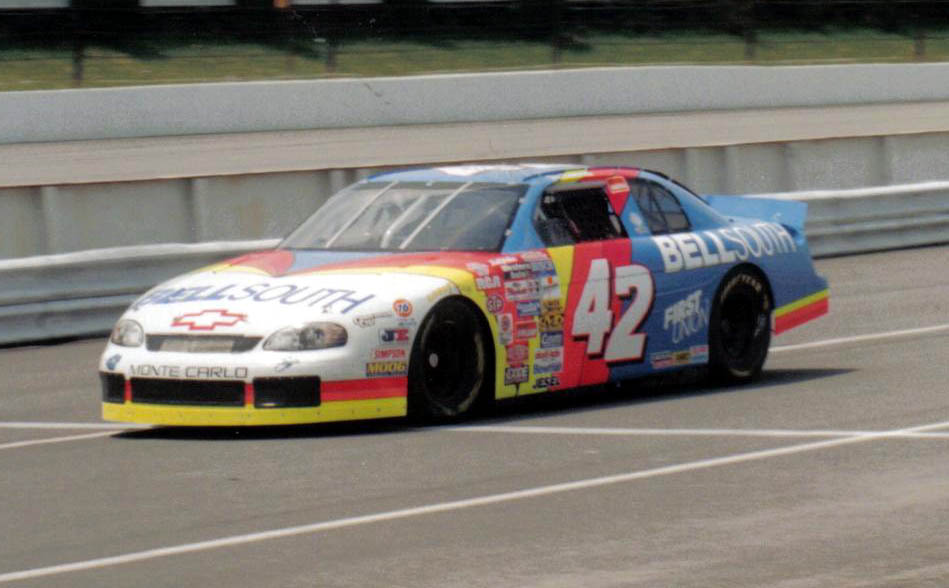The image captures a colorful, 90s-style NASCAR race car, predominantly painted in an eye-catching combination of white, yellow, red, and blue, parked on the side of a racetrack. The car's bold design features a blue rear, red diagonal stripes at the center near the driver's side door, a yellow section extending from the driver's door to the front wheels, and a white front. The car is adorned with the number 42 in large white numbers with a black shadow. Various sponsor logos, including Bell South, Monte Carlo, Chevy, First Union, RCA, and Jessel, are prominently displayed across the vehicle. The car's black tires have white writing around the edges. Metal bars, likely safety cages, are visible through the side windows and windshield. The car is positioned on a racetrack that has white lines and is bordered by a guardrail and concrete walls, with some grass visible beyond the enclosure at the top of the image.